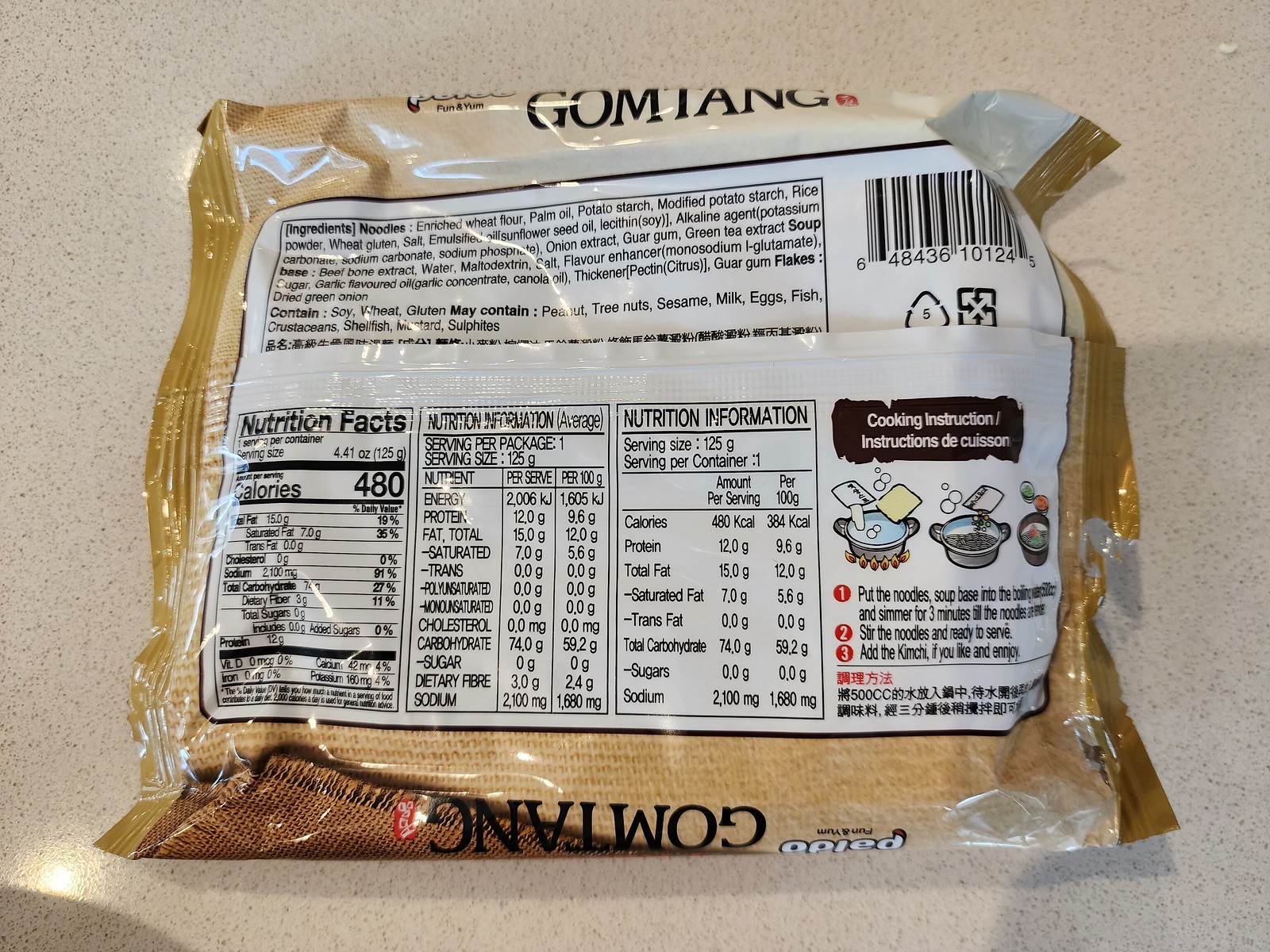This is a close-up, color photograph of the backside of a food package, specifically for instant ramen noodles named "Gumtang." The background is a beige, mottled color with various light and shadow gradients, creating a sense of depth. The package itself has a beige rim. Written at the top and bottom of the package is the brand name "Gumtang." 

Ingredients such as wheat flour, palm oil, potato starch, rice powder, onion extract, and beef bone extract are listed prominently at the top, supplemented by an allergy warning that indicates the presence of soy and wheat, and the potential for peanuts, tree nuts, sesame, milk, eggs, fish, crustaceans, shellfish, mustard, and sulfites being present. Beneath this is a line of text in an Asian language.

In the upper right-hand corner, there is a barcode accompanied by triangular and square symbols. The lower half of the image is dominated by nutrition facts spread across three different boxes, listing detailed nutritional information, including the total calories, which is 480. Cooking instructions can be found in a black rectangle at the lower left-hand corner, detailing the steps to prepare the noodles and soup base. Despite its detailed content, the package material seems akin to a sheet of cloth wrapped in plastic, ensuring the product inside remains protected.